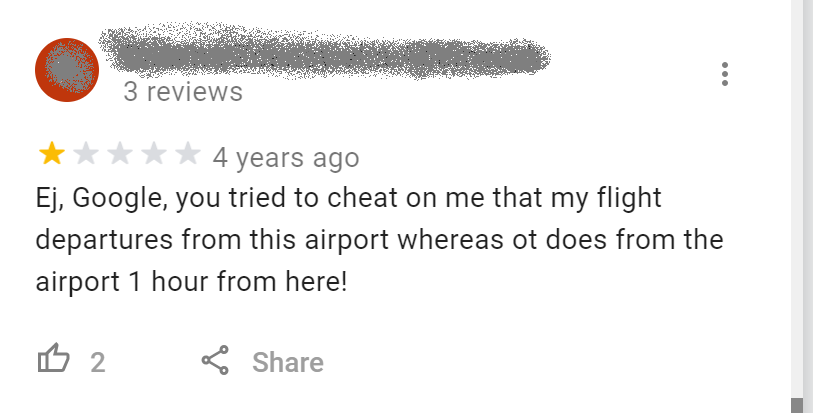The image is a heavily altered screenshot of a review displayed prominently on the top left corner. A striking red circle overlays the area, partially obscured by a bold spray of gray paint that covers the profile picture. The same gray paint also mists across the top portion, effectively blurring out the reviewer's name. Below this obscured section, three reviews are listed, but only one is visible. This review, posted four years ago by someone identified as "EJ" on Google, is starkly negative, rated at one out of five stars. The review text reads: "You tried to cheat on me that my flight departure from this airport whereas Ott does from the airport one hour from here," suggesting dissatisfaction with a flight service. The review has garnered two likes and features a share button underneath it. To the right of the image is a scrollbar, split into a light gray upper half and a darker gray lower half, contributing to the overall impression of a heavily edited and anonymized screenshot.